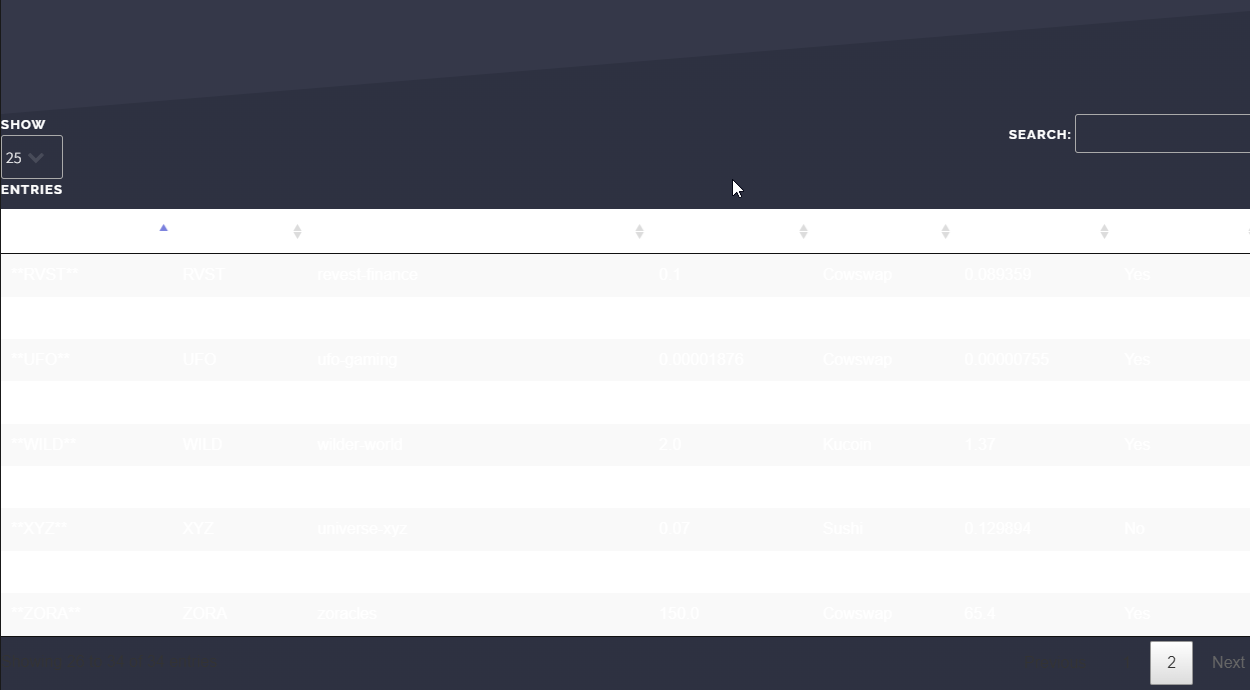This image is a screenshot of what appears to be the front page of an app. At the top left corner, there is a dropdown menu labeled "Show Entries" with the number 25 inside the selection box. On the top right side, a search bar is visible. The top header of the app is dark, possibly black, contrasting with the body of the page, which features a chart with a white background and white text, making it difficult to read.

Upon inspection, it seems that the first row of the chart reads "RVST" and "RVST" again, followed by the text "REVEST FINANCE," with numerical values such as "0.1" and "COWSWAP 0.089359". The chart comprises about 5 rows and either 7 or 8 columns. At the bottom corners of the screenshot, there are two buttons, one located at the bottom left and the other at the bottom right.

Overall, the white text on the white background significantly reduces the readability of the chart details, although some entries can be distinguished upon close examination.